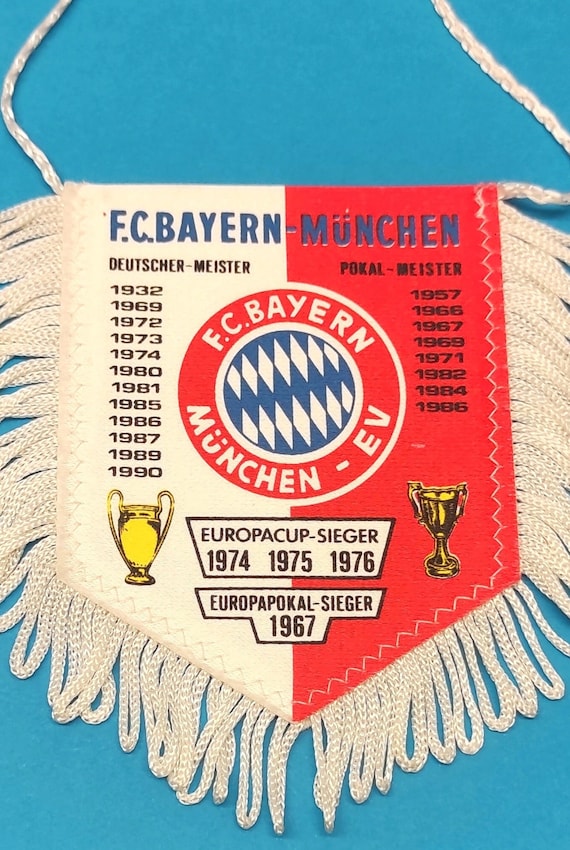The image depicts a hanging banner set on a baby blue table. The banner, representing the football club FC Bayern München, features a striking two-toned design: the left half is white and the right half is red. At the center of the banner is a prominent red circle inscribed with "F.C. Bayern." Inside this red circle is another concentric circle divided into blue and white diamond shapes, topped with "München eV." A looped white string extends from the top, suggesting it is designed to be hung. Along the edges of the banner, white fringe adds a decorative touch.

The banner is adorned with several inscriptions and illustrations of trophies, signifying various championship wins. On the left white section, under the title "Deutsche Meister" accompanied by a trophy, are the years 1932, 1969, 1972, 1973, 1974, 1980, 1981, 1985, 1986, 1987, 1989, and 1990. The right red section, labeled "Pokal Meister" and featuring another trophy, lists the years 1957, 1966, 1967, 1969, 1971, 1982, 1984, and 1986. Additionally, in black lettering, the banner marks "Europa Cup Sieger" with the years 1974, 1975, and 1976, alongside "Europa Pokal Sieger" for 1967.